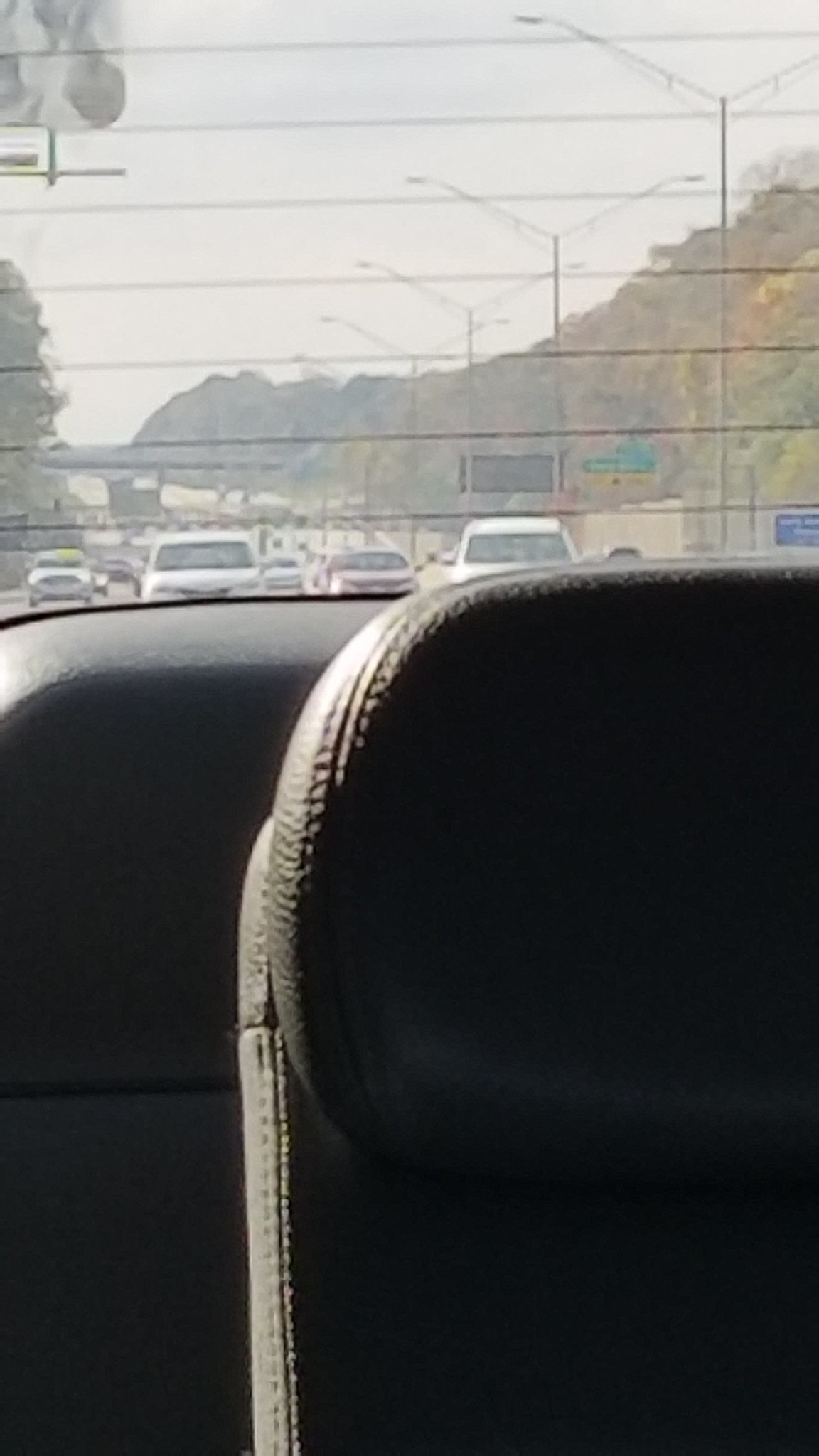The image captures a daytime highway scene from the back seat of a vehicle, looking out the rear window. The foreground shows the dark gray backseat and the interior rear panel, with horizontal defroster lines on the window. Outside, the highway stretches behind the car, curving slightly to the left. Several vehicles are visible, including a prominent white car and a red car. To the right, you see white poles with lights and a line of trees, extending towards the left. Hazy, rocky mountains form a gentle slope from the right. Traffic signs are present but indistinct due to the image's haziness. The overall impression is one of a busy multi-lane highway, viewed through the back window of a moving vehicle.